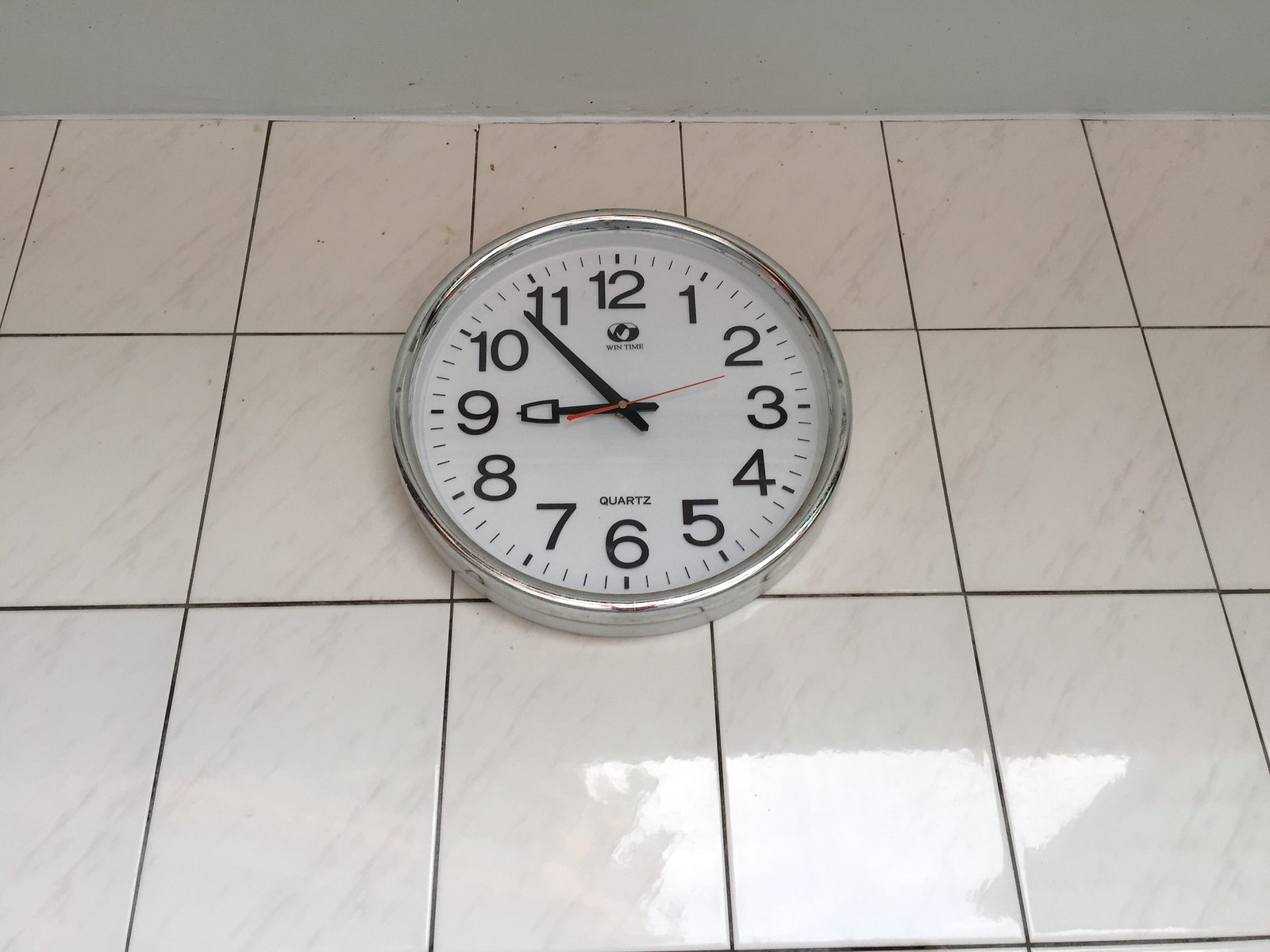In the image, a wall clock is prominently displayed, though it appears to be resting on a white, tiled floor that features subtle marbling. The background wall is a grayish tone, providing a stark contrast to the clock. The clock's face is a clean white with bold black numerals and the word "quartz" inscribed on it. The casing of the clock is a sleek silver. It shows the time at 8:53, with the black hour and minute hands pointing clearly, while the second hand stands out in red. Just beneath the 12 o'clock position, there is a logo that reads "[Something] Time," though the exact wording is indistinguishable.